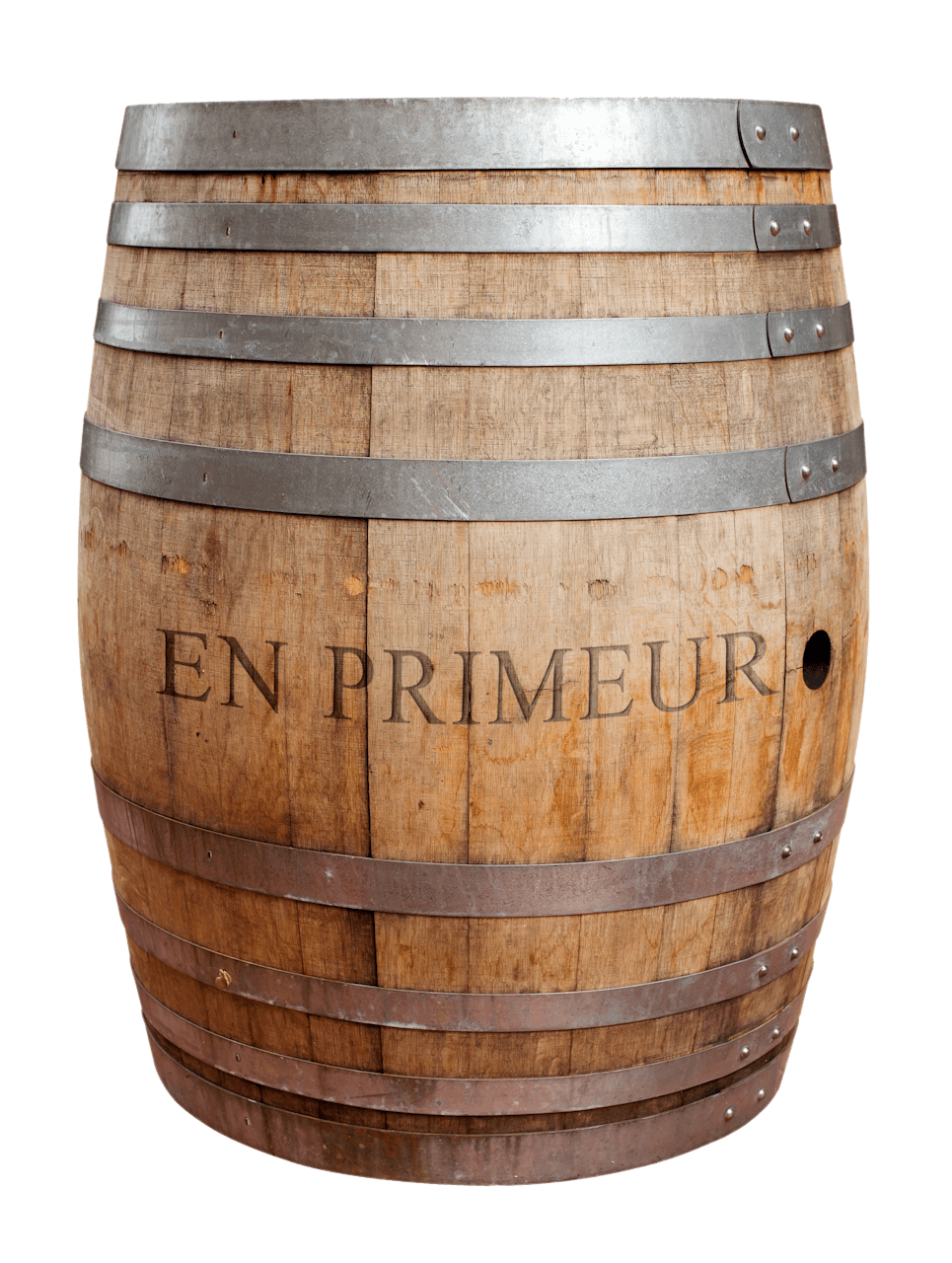This image depicts a rustic, aged wooden barrel set against a stark white background, suggesting a studio setting. The barrel features a mix of tan to dark chocolate brown wood tones that gradually fade from dark at the bottom to a lighter, unfinished look at the top. It is encircled by multiple silver metal straps or bands fastened with rivets, specifically four around the top and four around the bottom, spaced evenly along the circumference. An engraving in the center of the barrel reads "EN PRIMEUR," with a small black hole situated to the right of this text. The barrel’s weathered appearance, marked by signs of use, complements its overall antique charm. The studio lighting accentuates the right-hand side, adding depth and dimension to the detailed texture of the wood and metal.